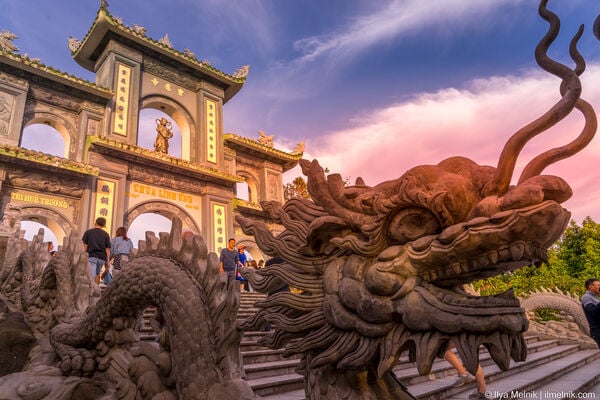This image depicts an intricately designed Chinese temple situated atop a hill, showcasing both historical and cultural significance. The temple features a series of ornate arches forming a shrine-like structure with a goldish statue at the center of its top tier. The roof is characteristically Asian, with pointed edges curving upward, and the structure is adorned with Chinese writing.

Descending from the temple, a long staircase made of gray concrete runs down the hill, guarded on either side by stone dragons. These dragons are highly detailed with scales, spikes, and fin-like whiskers surrounding their faces. Their mouths are open, revealing sharp teeth, and their large, expressive eyes enhance their imposing presence as they wind up the staircase like serpents.

The sky above is blue, punctuated with reddish and white clouds. Tourists can be seen climbing the stairs, adding a sense of scale and activity to the scene. The intricate architecture and the majestic dragons highlight the grandeur of this outdoor monument, while green leaves and the name 'Aya Melnik' in white text add subtle details to the composition.